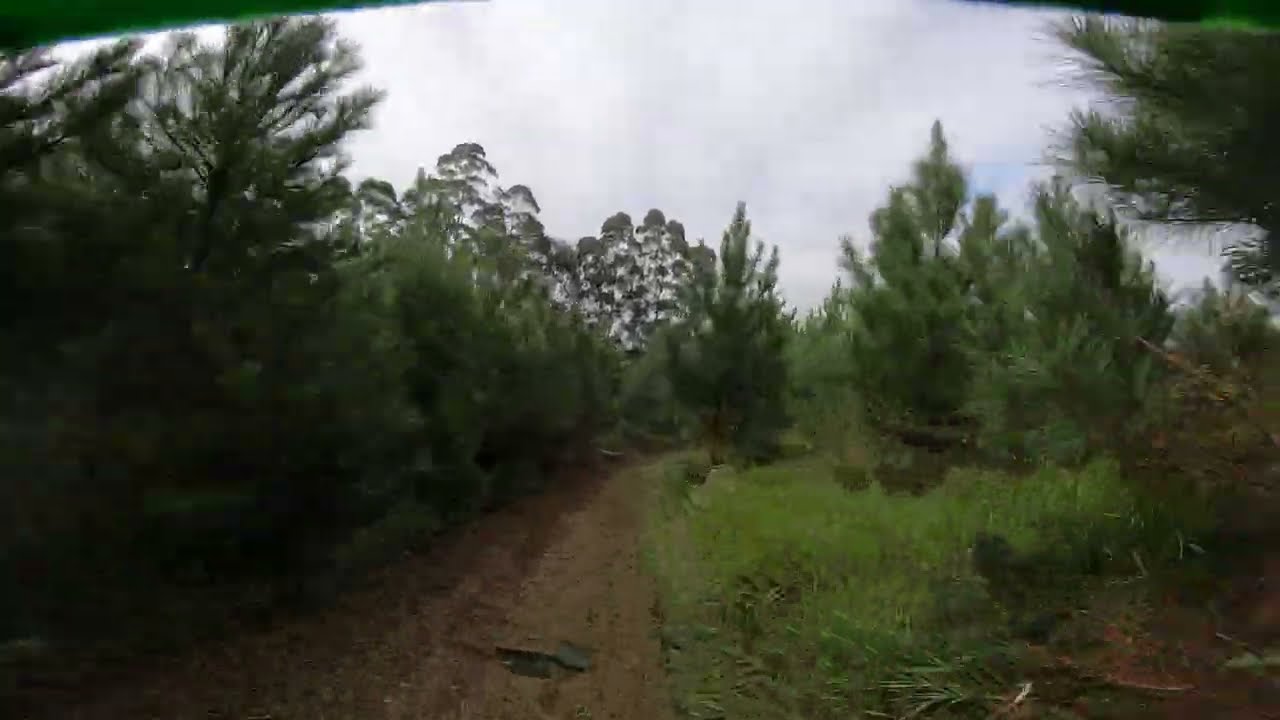The image captures a narrow dirt path winding through a secluded, heavily wooded area predominantly featuring pine trees on both sides. The path appears to be about four feet wide and is partially obstructed in the distance by a fallen tree or dense foliage, obscuring the view of what lies beyond. Flanking the trail, there are patches of green grass mixed with areas of bare earth and pine needles. The weather is overcast, with a gray, cloudy sky that shows only hints of blue but no direct sunlight or rain. The perspective of the photo suggests it was taken from someone riding a bicycle or motorcycle, likely equipped with a GoPro camera, as the edges of the image show some curvature typical of a helmet-mounted camera. The foreground displays a pothole on the left side of the path and indicates motion, as the blur on the grass at the path's edge implies the scene was captured at a speed faster than walking. In the background, some eucalyptus trees are discernible among the dense pine grove.